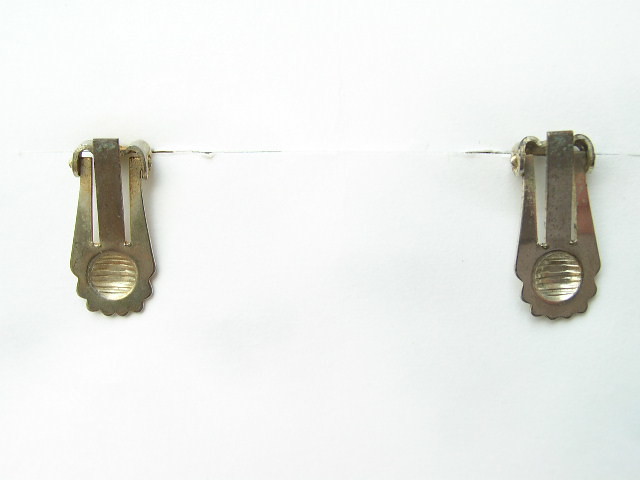This photograph showcases a pair of eye hooks mounted on a pristine white wall, seemingly part of a larger white surface or box. These hooks, made of brass with a gold finish, exhibit signs of age, including a touch of rust at the top. Each eye hook features a concave circle at its base resembling a round face without distinct facial features, which then transitions into a vase-like shape. The hooks are adorned with a floral pattern at the lower end, consisting of half circles forming petal-like edges and a dimpled center with intricate ribbing. Alongside the hooks, there is a noticeable line or seam on the wall, possibly indicating damage or a join in the panels. The hooks, secured with crimped extensions, add a vintage yet functional aesthetic to the surface they are fastened to.